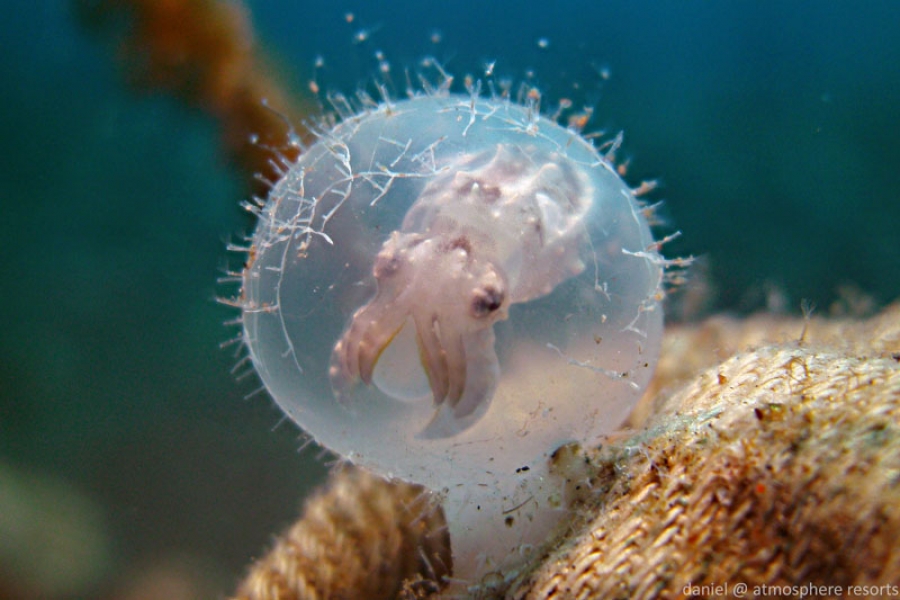The photograph showcases a detailed close-up of a pink, translucent octopus or squid-like creature encased in a somewhat translucent egg sac. Within the egg, the creature's multiple tiny tentacles and two distinct eyes are visible, suggesting its small size and early developmental stage. The egg sac has fine, hair-like structures around its edges, anchoring it to an orangish surface that might be rock or coral. The seafloor environment in the background is blurred, hinting at underwater vegetation such as seaweed. In the bottom right corner, the image is marked with a white watermark that reads "Daniel at Atmosphere Resorts," indicating the photograph's origin.